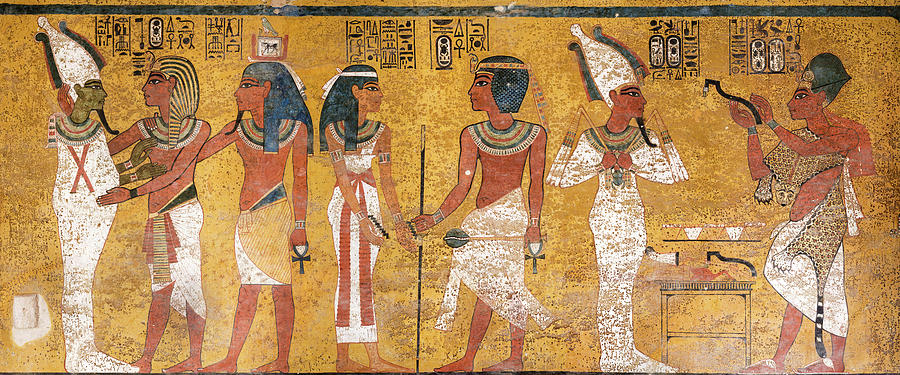This captivating color photograph showcases a rich tableau of ancient Egyptian wall art set against a luxurious gold-background. At the top, hieroglyphics are elegantly inscribed, adding an authentic touch to the scene. The wall art features seven distinct Egyptian figures, each adorned in traditional attire and positioned in a compelling narrative sequence.

From left to right, we first encounter a standing mummy with its brown hands extending forward. Adjacent to the mummy is a man clad in a sarong and a long beaded necklace, followed by another man similarly dressed but distinguished by the Egyptian ankh he holds. Moving right, a woman exudes grace in a lovely white gown, her arms decorated with bangles and her long black hair crowned by a beaded necklace.

Next to her stands a younger man, whose details blend into the collective elegance of the tableau. Beside him, a figure initially mistaken for a woman due to the adornments, is revealed to be a man dressed in a pristine white outfit from head to toe, complemented by a pointed hat and a long black beard. He holds an object in each hand, suggesting a spiritual or ritualistic role.

Finally, at the far right, stands a figure robed in leopard skin with a white robe underneath, grasping a black object, possibly a snake. This arresting depiction of seven diverse figures in ancient Egyptian attire against a gold backdrop, enriched with hieroglyphics, offers a mesmerizing glimpse into the storied past of Egypt.